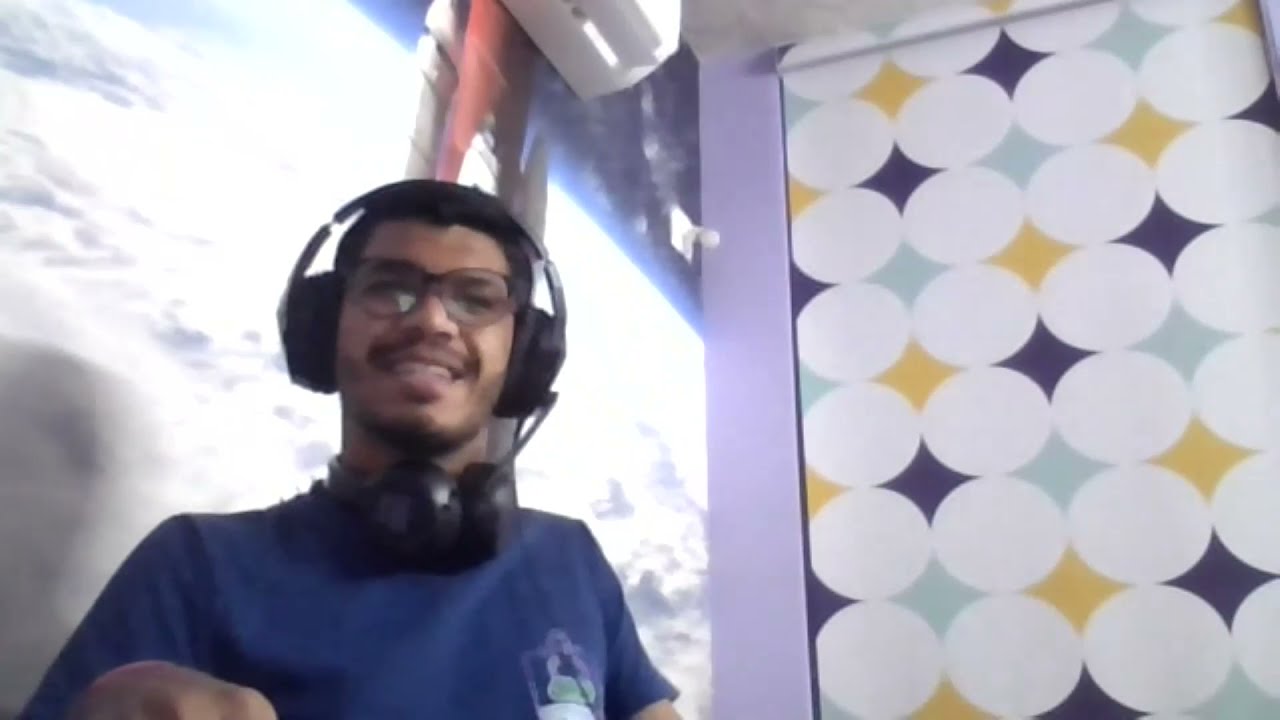The image depicts a man of possibly Indian descent, with a darker complexion, situated on the left side of the frame, looking down towards the camera. The camera angle suggests the perspective from a laptop placed on a table, angled upwards. He is dressed in a dark blue t-shirt and wears medium-framed black glasses. His short black hair and black stubble are visible. He is smiling broadly, revealing his teeth. Remarkably, he has two headsets: one large, over-ear black headset on his head, and another headset resting around his neck like a collar. The image background features two distinct sections: one side showcases a wall with an image or painting of a red and white rocket launching from Earth, set against a sky or outer space backdrop. This section also includes a peek of an air conditioning unit at the top. The other side presents a light purple wall adorned with a polka dot design featuring white, blue, green, and yellow stars. The photograph is slightly grainy, suggesting it might be a screenshot from a video. The overall lighting is bright and natural, enhancing the vividness of the various colors in the scene.